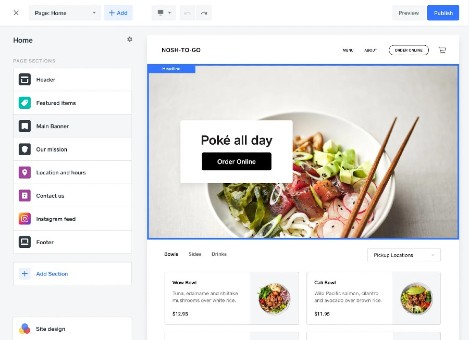The screenshot features a predominantly gray background, with various interactive elements and sections clearly indicated. 

At the top, there are two buttons: one labeled "Preview" on a gray rectangle, and another labeled "Refresh" on a blue rectangle. To the left, navigation icons include "Home," a settings icon, and "Page Settings." Below this, a list is displayed, and at the very bottom of the screen, there is an "Add Section" button with a blue square containing a plus symbol.

In the center, there is a header labeled "nosh2go" (spelled N-O-S-H), accompanied by a shopping cart icon on the right. Below this header, there is an image that appears to feature an assortment of vegetables alongside a pair of chopsticks.

Further down, there is a text section titled "Poke All Day," with the subtitle "Order Online" in white text on a black rectangle. Below this title, categories listed include 'Bowls,' 'Sides,' 'Drinks,' and 'Pickup Location.' Currently, two images are displayed as part of the content.

The visual elements are organized into various shapes and colors, including a prominent 'X,' a gray rectangle, a blue rectangle, and three gray squares, contributing to the structured layout of the interface.